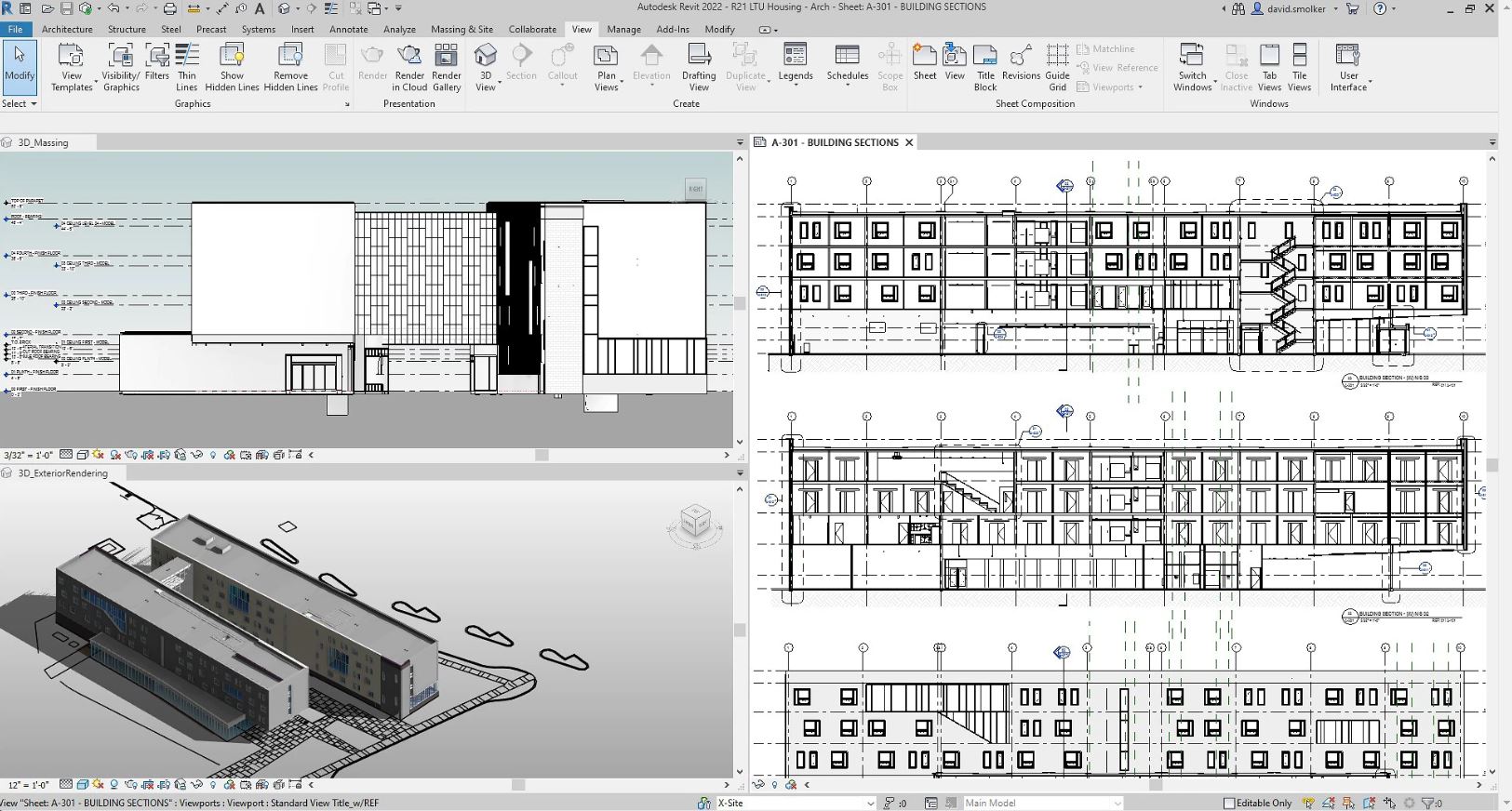Davis Smucker is working on architectural blueprints displayed on a computer screen. The software's interface at the top features various menu options including File, Modify, Architecture, Structure, Still, Precast, System, Insert, Antidote, Analyze, Mass and Incite, Collaborate, View, Manage, Add, and Modify. Control icons for Minimize, Assemble, and Exit are also visible. The screen shows detailed blueprints of a three-level building on the right side, rendered in gray and white tones. In the lower left corner, there is a section labeled "Sheet A-301" which includes additional details such as "Building Sections," "Viewpoint," "Standard View," and "Title."